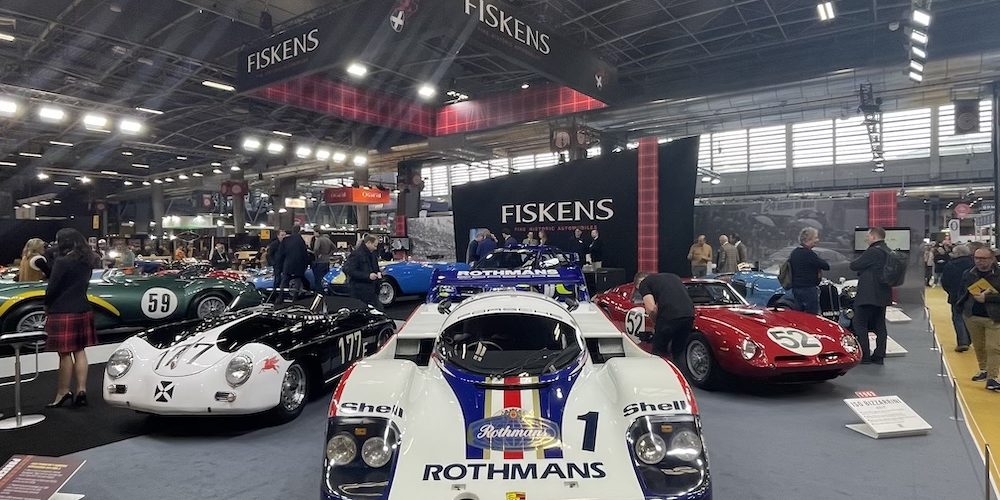The image depicts an expansive auto show held in a large warehouse-like garage, buzzing with activity. The ceiling is adorned with various artificial lights, and natural light also filters in through a large window in the background. Central to the image is a striking white racing car, prominently displaying the brands "Shell" and "Rothmans" on its hood, along with a distinctive blue, red, and white stripe. This car is marked with the number 1. Surrounding it, several other sporty cars catch the eye, including a red car with the number 52, a white car with the black number 177, and a green car bearing the number 59. A billboard with "Fiskens" written in large white letters dominates the scene, clearly indicating the event's sponsor. Below, a short fence separates curious onlookers from the vehicles. Many people are milling about, some admiring the cars up close, others engaging in conversations, and a few appearing to conduct interviews. Among the crowd, diverse attire stands out, including a person in a red and black plaid skirt and another couple dressed mostly in black.